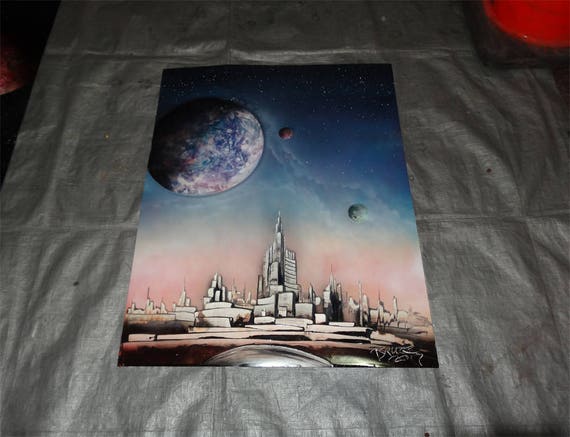The image showcases a vertically oriented poster resting on a gray painter's cloth spread over a bed. Dominating the poster is a depiction of a futuristic cityscape set against a celestial backdrop. The city features tall, white stone buildings, with a central structure rising above the others. The scene is framed by an Earth-like planet in the top left, its blue and white hues suggesting a partially frozen surface. Beside it, two more planets float: a brown one close to the Earth-like planet and a smaller, light bluish-green one further down to the bottom right. The sky above the city transitions from dark black-blue, scattered with stars and planets, to a light pinkish horizon encircling the cityscape below. An orange traffic cone is positioned in the upper right corner outside the poster, near a black square base, adding an unexpected element to the scene. The overall artwork combines elements of realism and representationalism, creating a vivid and imaginative portrayal of an otherworldly city.